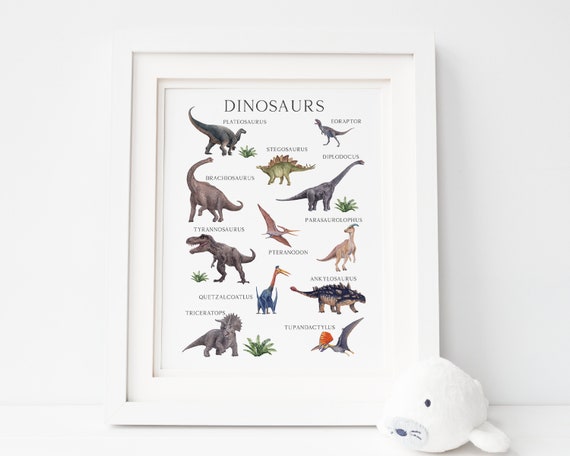This indoor photograph captures a framed art piece, ideal for a child's room. The artwork, set against a white wall, appears to be either on a white mantelpiece or floor. It features a white frame and matting. Bold black letters at the top spell out "Dinosaurs," beneath which are colorful illustrations of approximately 10 to 12 dinosaur species, including a Platysaurus, Stegosaurus, Triceratops, and Tyrannosaurus. The dinosaurs are evenly spaced across the white background, each accompanied by a text label identifying the species. In the bottom right corner of the image, a plush white stuffed toy, resembling a seal, adds a cozy touch to the scene. The overall palette of the photo is primarily white and gray, with the vibrant dinosaur illustrations providing the main bursts of color.